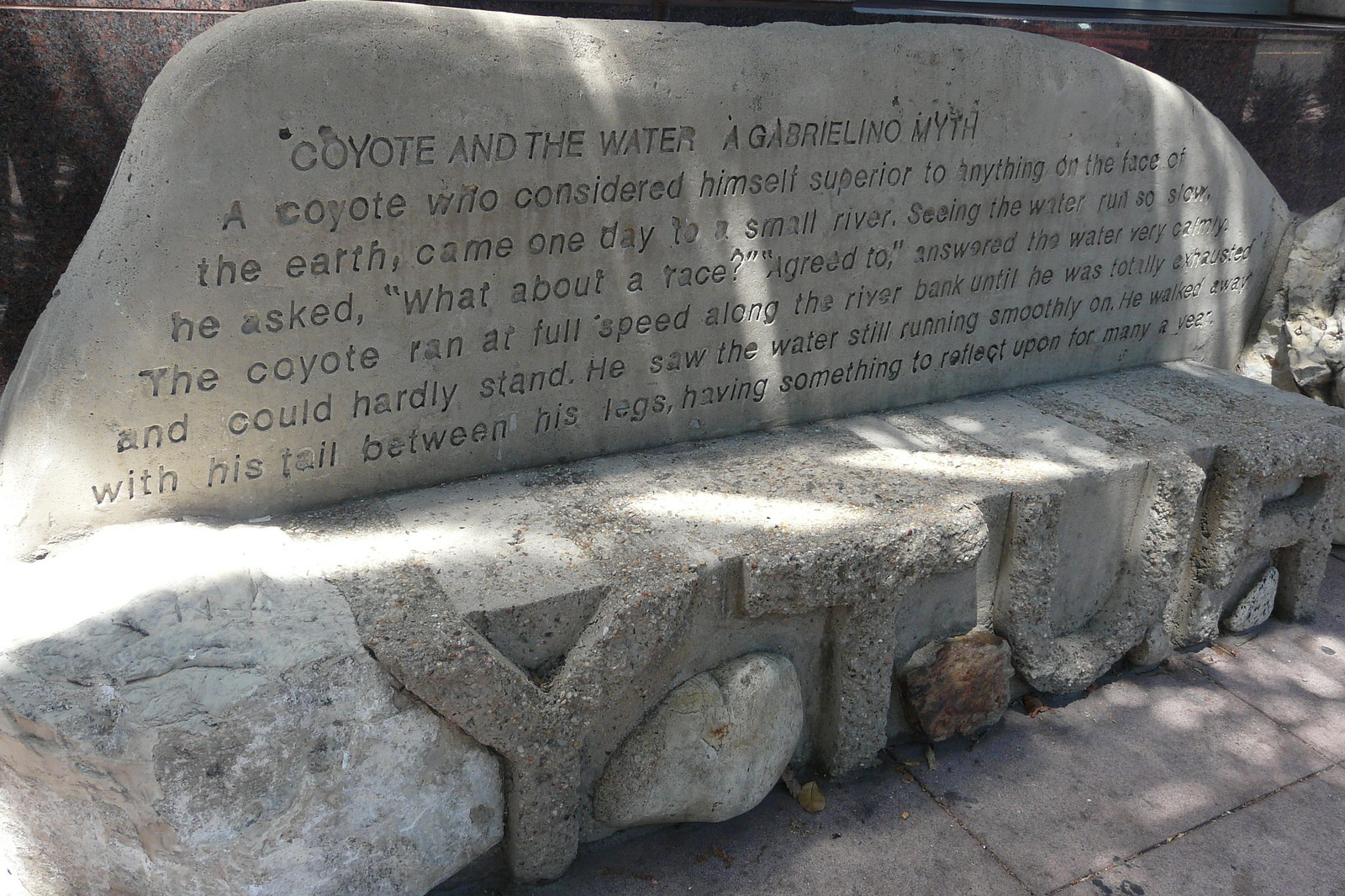The image showcases a large carved stone bench made entirely of concrete and stone. The backrest of the bench features an engraved paragraph that narrates a Gabrielino myth titled "Coyote and the Water." The story describes a coyote named Wilo who considered himself superior to everything on Earth. One day, he came across a small river and, noticing the water running slowly, challenged it to a race. The water calmly accepted. The coyote ran at full speed along the riverbank until he was completely exhausted and could barely stand, while the water continued flowing smoothly. Humiliated, the coyote walked away with his tail between his legs, left to ponder his experience for many years. Below the story, the bench also displays the letters "Y-T-U-R." The image captures this scene during the daytime, highlighting the detailed engravings and the stone material of the bench.